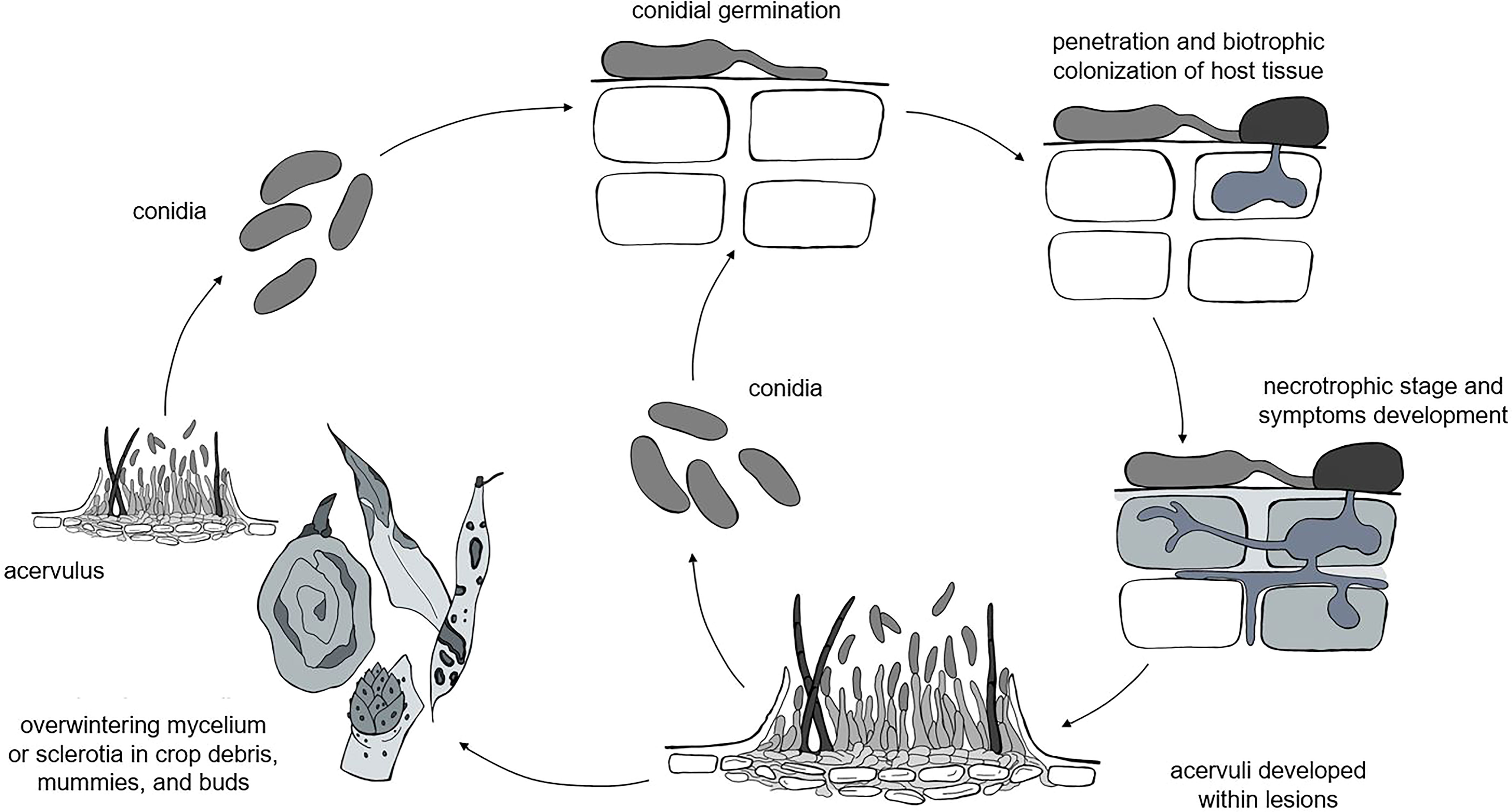The image presents a detailed flowchart illustrating the life cycle of a pathogenic organism. This cycle begins with "Conidial Germination," depicting a long, skinny creature preparing to penetrate the host. Next, it moves to "Penetration and Biotrophic Colonization of Host Tissue," showing a smaller, rounder bean-like creature being penetrated by a longer, narrower organism, depicted with underground root-like structures. The cycle progresses to the "Necrotrophic Stage and Symptoms Development," where the penetrating creature injects substances into the host, leading to the growth of gray root-like structures.

This stage is followed by "Acervuli Developed Within Lesions," showing skin-like cells with long, narrow projections, above which the conidia (small bean-like creatures) are illustrated. These conidia return to the top of the cycle in the "Conidial Germination" phase. Alternatively, the cycle can branch out to "Overwintering Mycelium or Sclerotia in Crop Debris, Mummies, and Buds," which features geometric, leaf-like shapes. The process eventually circles back to the conidial stage, depicting how the cycle perpetuates.

The prominent colors in the image are black, white, and gray, with each stage clearly illustrated through small diagrams that resemble seeds or beans transitioning through various forms at each stage of the cycle.